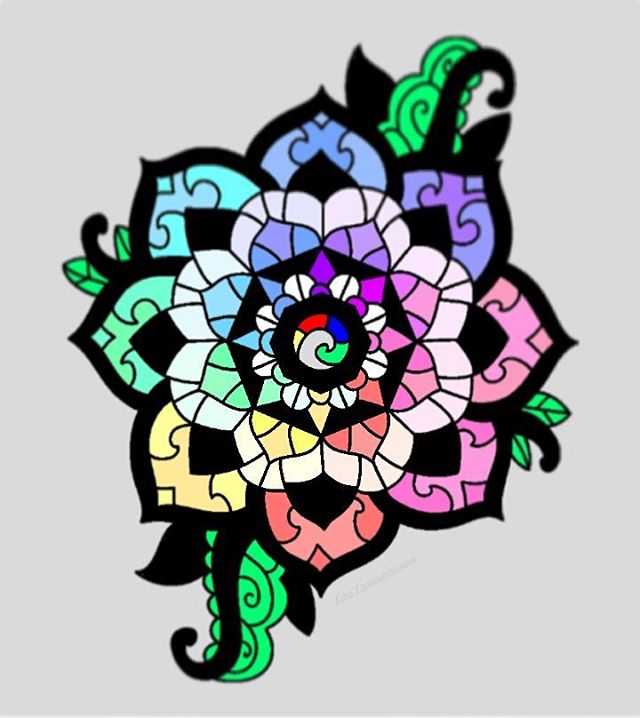The image portrays an intricately detailed drawing resembling a stained glass artwork, set against a light gray background. Dominating the composition is a flower-like shape with pointy petals radiating outward in a harmonious array of vibrant colors including pink, orange, yellow, green, and various shades of blue. Each petal is distinctly outlined in bold black lines, giving the piece its stained glass effect. The flower is multi-layered, featuring a core layer of white petals encircled by additional layers of colorful petals in blue, green, yellow, and orange hues. Decorating the sides of the flower are lush green leaves and winding black tendrils, which add an organic touch to the geometrically structured petals.